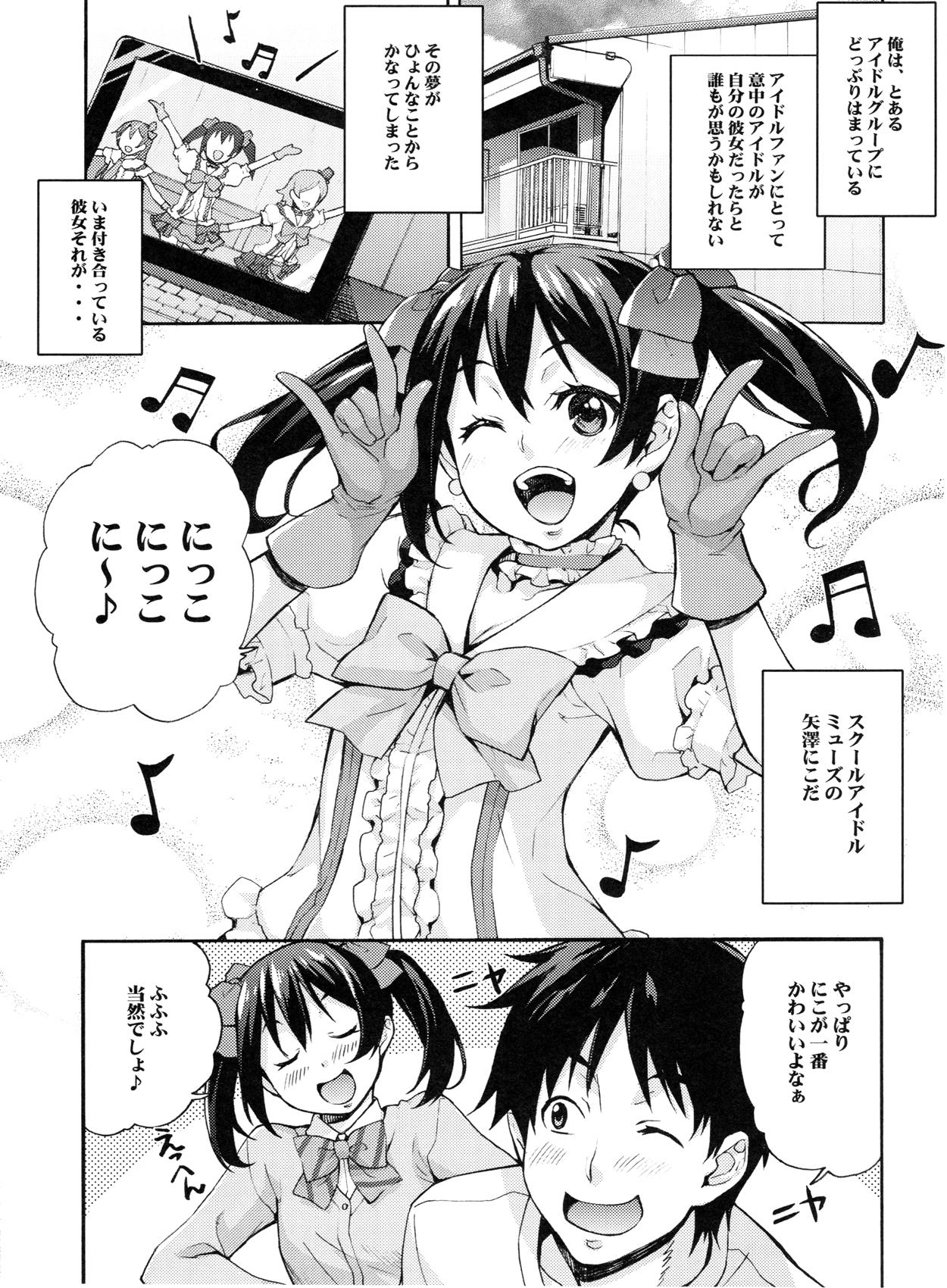This hand-drawn, detailed Japanese comic showcases several vibrant scenes. In the top left corner, a laptop screen displays three girls energetically dancing and singing. The girl in the middle strikes a V-shape pose with her arms, flanked by the girls on either side holding hands, surrounded by music notes. The top right corner captures a view of a house’s second floor, complete with a balcony and an open door leading to it. The central image focuses on a jubilant girl with pigtails adorned with large butterfly bows, one on each side and another on her chest, striking a celebratory pose with her arms up and a wink, enveloped by musical notes. Below, in the final scene, the same girl, with her eyes closed and mouth open in joy, stands next to a boy who has one eye closed and the other open, engaging in a spirited conversation. Each panel is interspersed with Japanese text, adding depth to the lively narrative.